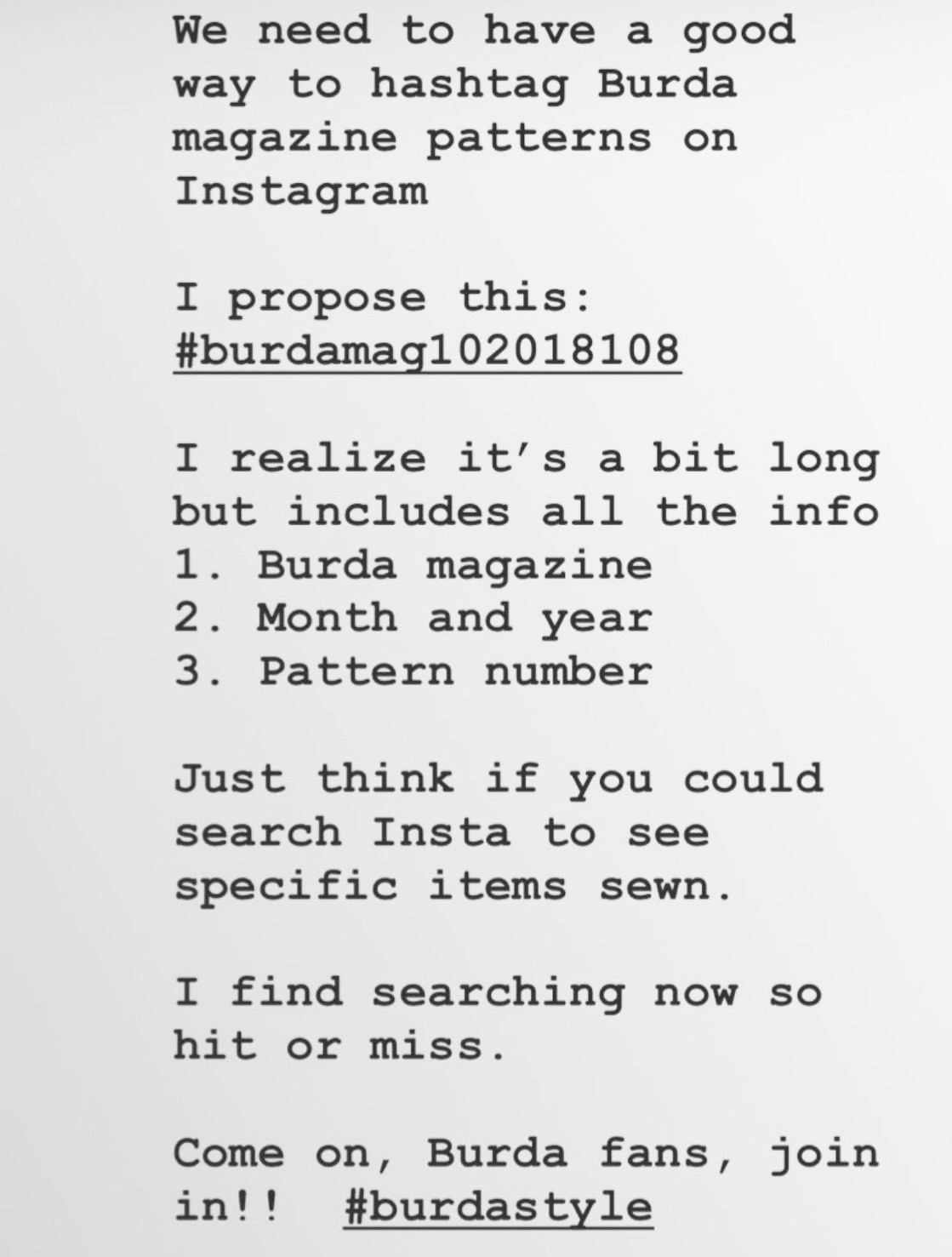In the image, black text is set against a plain white background, centered and taking up most of the visual space, presented in a standard Times New Roman font. The message advocates for a standardized method to hashtag Berta Magazine patterns on Instagram, suggesting the use of #BertaMag102018108. Despite acknowledging the length of the hashtag, the text argues it includes essential details: Berta Magazine, the month and year, and the pattern number. The text highlights the inconsistency of current search results and encourages Berta fans to adopt the proposed hashtag to streamline the search process on Instagram. The overall composition resembles a large block of text, akin to a social media post, drawing viewers' attention to the need for an organized hashtag system.